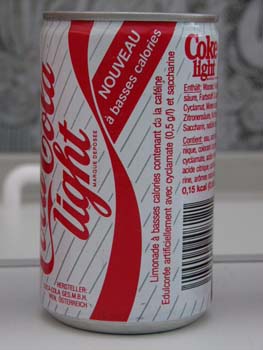The image depicts an unusual version of a Coca-Cola can, notably different from the classic red design with white lettering. This can is primarily white, adorned with thin diagonal silver lines that allow the aluminum background to subtly show through, creating a sleek and modern look. The aluminum body appears thicker, giving it a sturdier appearance. The text on the can reads "Coca-Cola Light" in the iconic Coca-Cola script, with the word "Light" written in lowercase. 

A distinctive red swoosh runs along the side of the can, and a small, sideways banner featuring the word "Nouveau" and the term "Calorie" suggests this is a French variant of the beverage. The term "Nouveau" indicates it might be a new edition. Above the "A" in "Calorie," there's a circumflex accent, hinting that this product could be marketed as low-calorie. 

The rest of the text on the can is too small to discern, but it appears bilingual, likely in both English and French. A partial view of the UPC code is visible, though the numbers are obscured due to the can's orientation. The can is placed on a white surface, with a white shape that resembles a cabinet handle in the background. The top part of the background seems to be patterned wallpaper, adding a subtle texture to the overall scene.